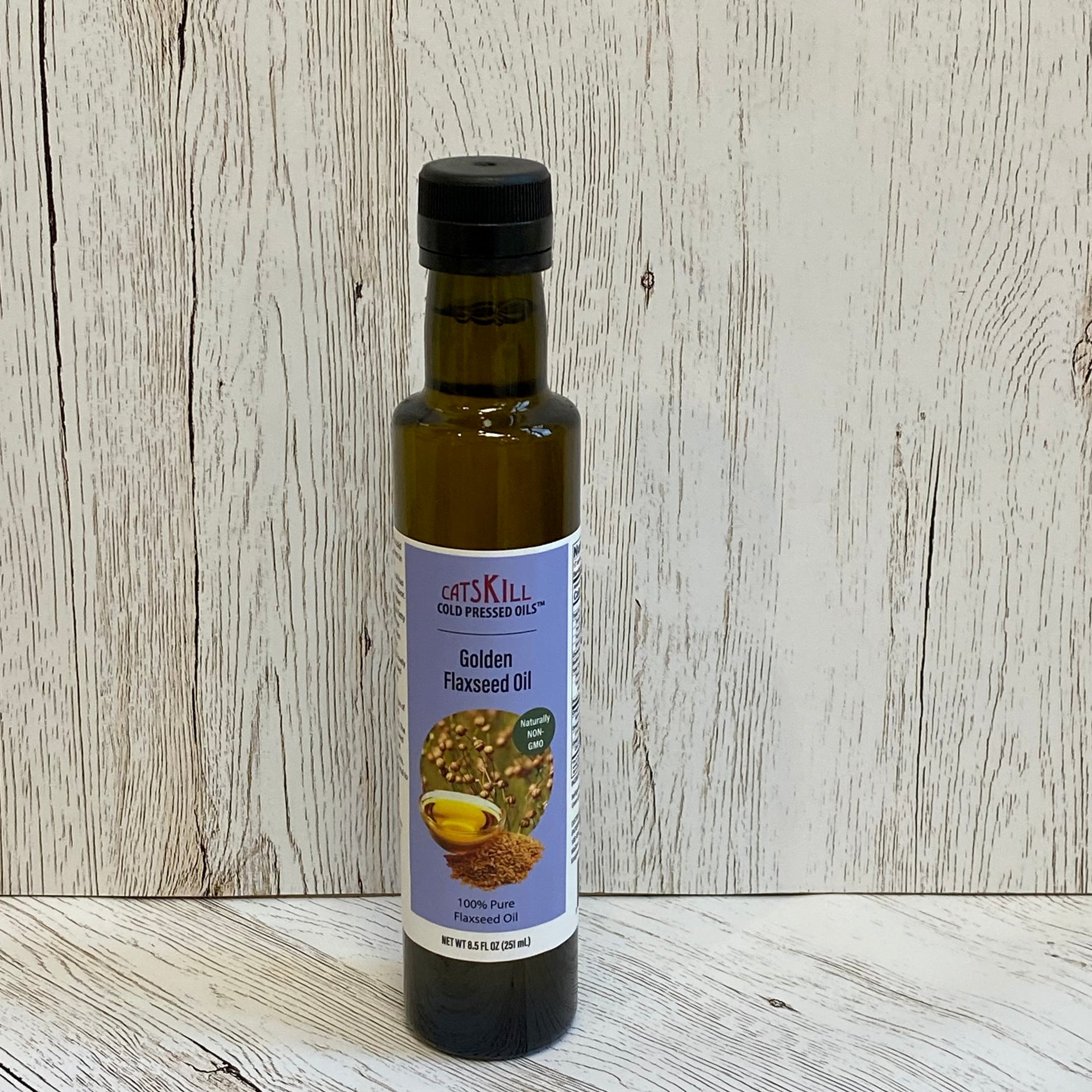This image features a slender, shiny, dark brown glass bottle with a black plastic twist cap. The bottle is adorned with a light lavender label bordered with white. At the top of the label, in red text, it reads "CATSKILL," followed by "cold pressed oils" in black text beneath. The product name, "Golden Flaxseed Oil," is prominently displayed in bold black text under a horizontal rule. A circular illustration depicting a brown flaxseed plant with bulbous ends, a small bowl of yellow liquid likely representing the oil, and a small pile of flaxseeds is centrally positioned on the label. Adjacent to this illustration, a green badge declares "Naturally Non-GMO." Near the bottom of the label, it states "100% Pure Flaxseed Oil" along with the net weight of 8.5 fluid ounces. The bottle itself is set against a light beige, wood-grained tabletop, which complements the label’s colors and highlights the overall presentation.